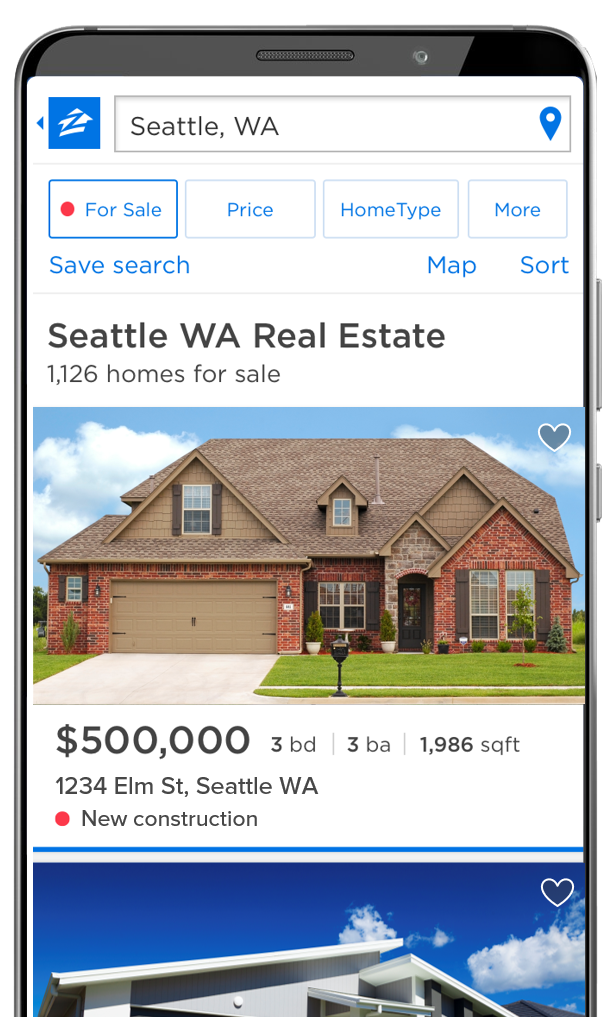The image displays a cell phone featuring the Zillow app. The phone itself has a black interior border with a silver exterior edge. On the right side of the phone, there is a volume control button positioned about three-quarters of the way up, with a power button slightly below it. The top of the phone showcases an area for the speaker and front-facing camera against a white background.

In the upper left corner of the app interface, there is a blue box with a house icon and a blue "Z" inside it. Below this, a search bar reads "Seattle, Washington" with a blue pinpoint icon next to it. The interface offers four selectable options: "For Sale," "Price," "Home Type," and "More," with the "For Sale" option marked by a red dot. Additional buttons include "Save Search," "Map," and "Sort."

The main section of the screen shows two property images. The lower image features a house with a blue sky backdrop, partially cut off. The middle section lists "Seattle, Washington real estate, 1,126 homes for sale" and highlights a property with a red brick building and a brown tiled roof. Detailed information for this property includes: $500,000, three bedrooms, three baths, 1,986 square feet, located at 1234 Elm Street, Seattle, Washington, labeled as "new construction." A favorite heart icon appears in the upper right corner of this property listing.